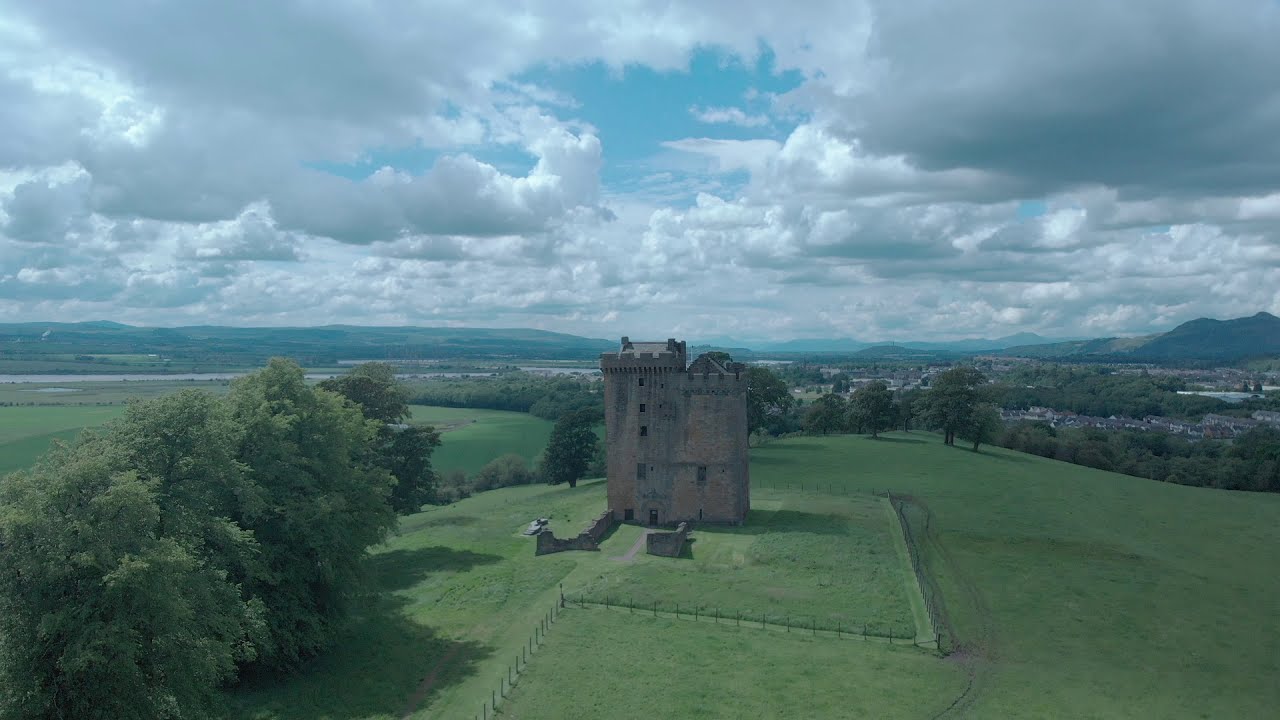This high-altitude drone shot captures a striking aerial view of a towering, medieval-style building, reminiscent of a castle with its crown-like roof edges. The beige brick structure, standing approximately forty feet tall, is centrally positioned in an expansive, verdant grass field. Surrounding the building, a fence is visible, enclosing the castle-like structure. The lush green field is framed by clusters of trees, particularly noticeable in the bottom left and along the edges of the photograph. In the distant background, a body of water, likely a lake or river, adds depth to the scenery, and farther back, there appears to be a small town with modern buildings. The sky above is filled with a variety of clouds, contributing to the overcast ambiance of the scene. The image is rich in color, featuring hues of green, blue, gray, tan, brown, black, and white, and conveys a historical yet tranquil outdoor setting with a blend of natural and architectural elements.